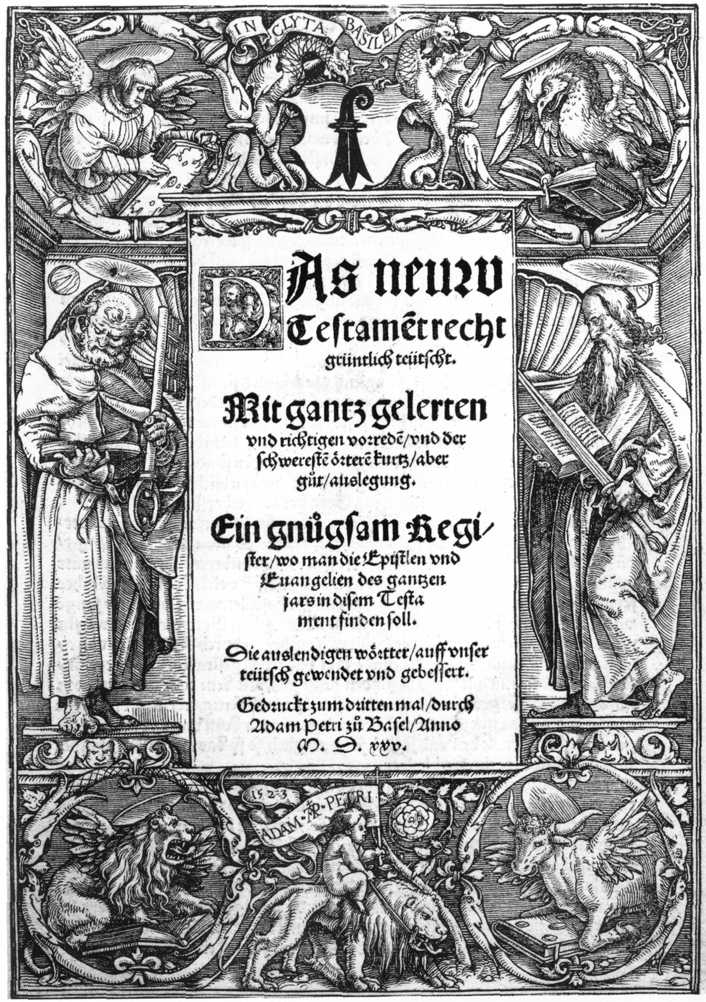The image is a black and white illustration of a 16th-century woodcut titled "Tidal Plate with St. Peter and St. Paul," created by Hans Holbein the Younger in 1523. This intricate illustration, primarily in portrait orientation, features a composition that evokes a religious and heraldic theme possibly resembling a coat of arms. In the central panel, Gothic typography in German adorns the piece, with an illuminated manuscript-style initial cap situated at the top left.

Dominating the center are two saintly figures, likely St. Peter and St. Paul, one holding a scepter and the other a sword and scripture. Surrounding them are various circles depicting religious settings in each corner. The top left corner presents an angel with wings, a halo, and a tablet, while the top right features an eagle with a halo reading a book. The bottom right corner shows a winged cow with horns kneeling before a book, and the bottom left showcases a lion with wings also in front of a book. Additionally, at the bottom center, there's an image of a man riding a lion with a banner overhead. The entire artwork is set against a gray background, enhancing the woodcut's detailed engraving style that exemplifies the Northern Renaissance aesthetic.